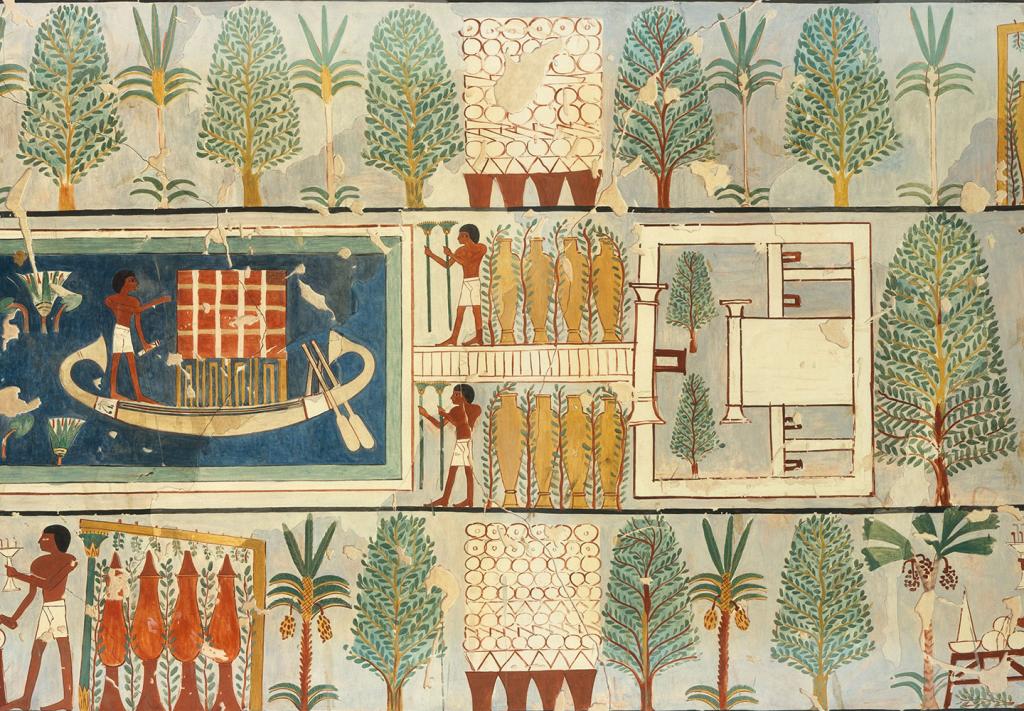The image depicts an ancient Egyptian painting divided into three horizontal panels. The top panel features alternating date palms and leafy green trees against a gray background, encapsulating elements of nature central to Egyptian culture. The middle panel showcases a vibrant scene set on blue water, highlighting a boat with a red roof and a dark-skinned man in white shorts. He holds two green poles suggestive of ceremonial lamps, surrounded by ceramic urns. The bottom panel repeats the presence of ceramic urns alongside more trees, grounding the composition in both botanical and human activity. The simplistic yet colorful depiction includes key Egyptian elements such as people standing in profile, underscoring classic stylistic traditions.